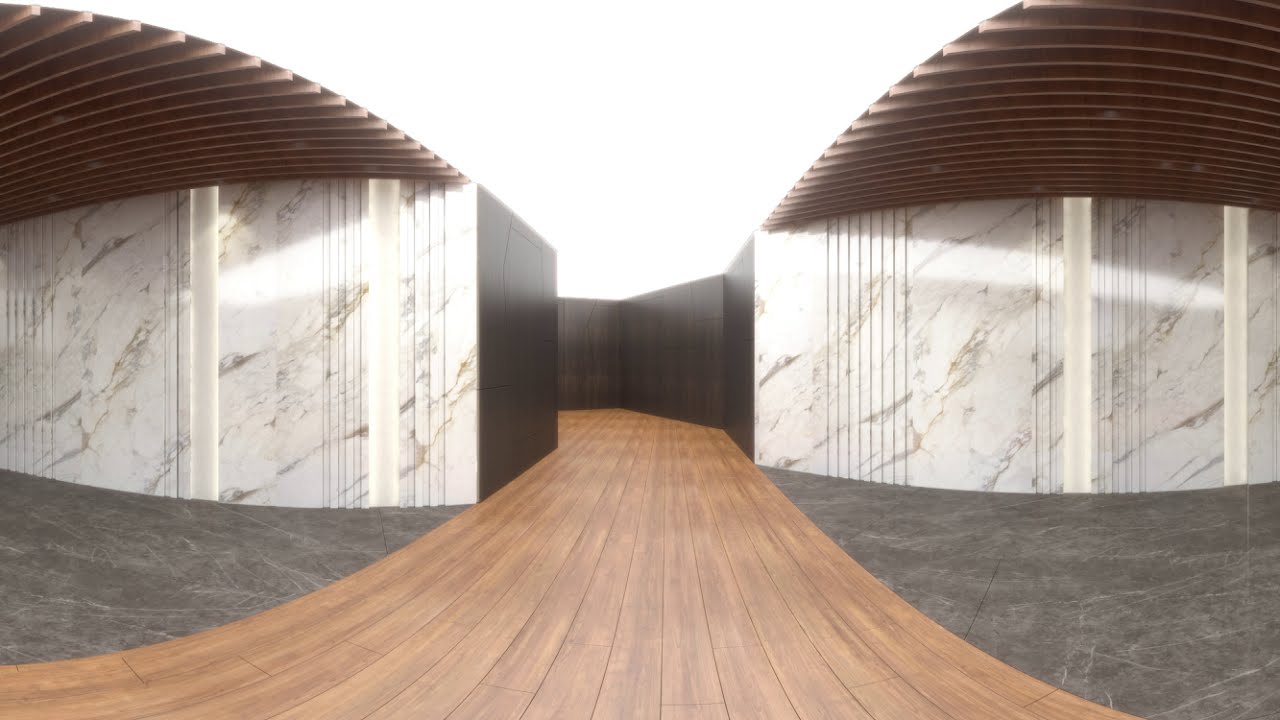In the image, a wide wooden walkway of light to medium brown wood starts at the bottom center and stretches towards the middle of the frame. Flanking this walkway on either side are dark marble floorings with white veining, offering a stark contrast. The walls adjacent to this pathway are composed of light-colored marble, also veined with gray, adding a sophisticated texture to the scene. Above, a ridged brown ceiling made of rafters or wooden beams frames the top of the image, while the upper center section displays a bright white, V-shaped area, suggesting an exterior light source. Despite the outdoor-like brightness at the top, the rest of the setting appears semi-enclosed, with an ambiance that blends both interior and exterior elements. The overall color palette includes whites, dark browns, lighter browns, and grays.